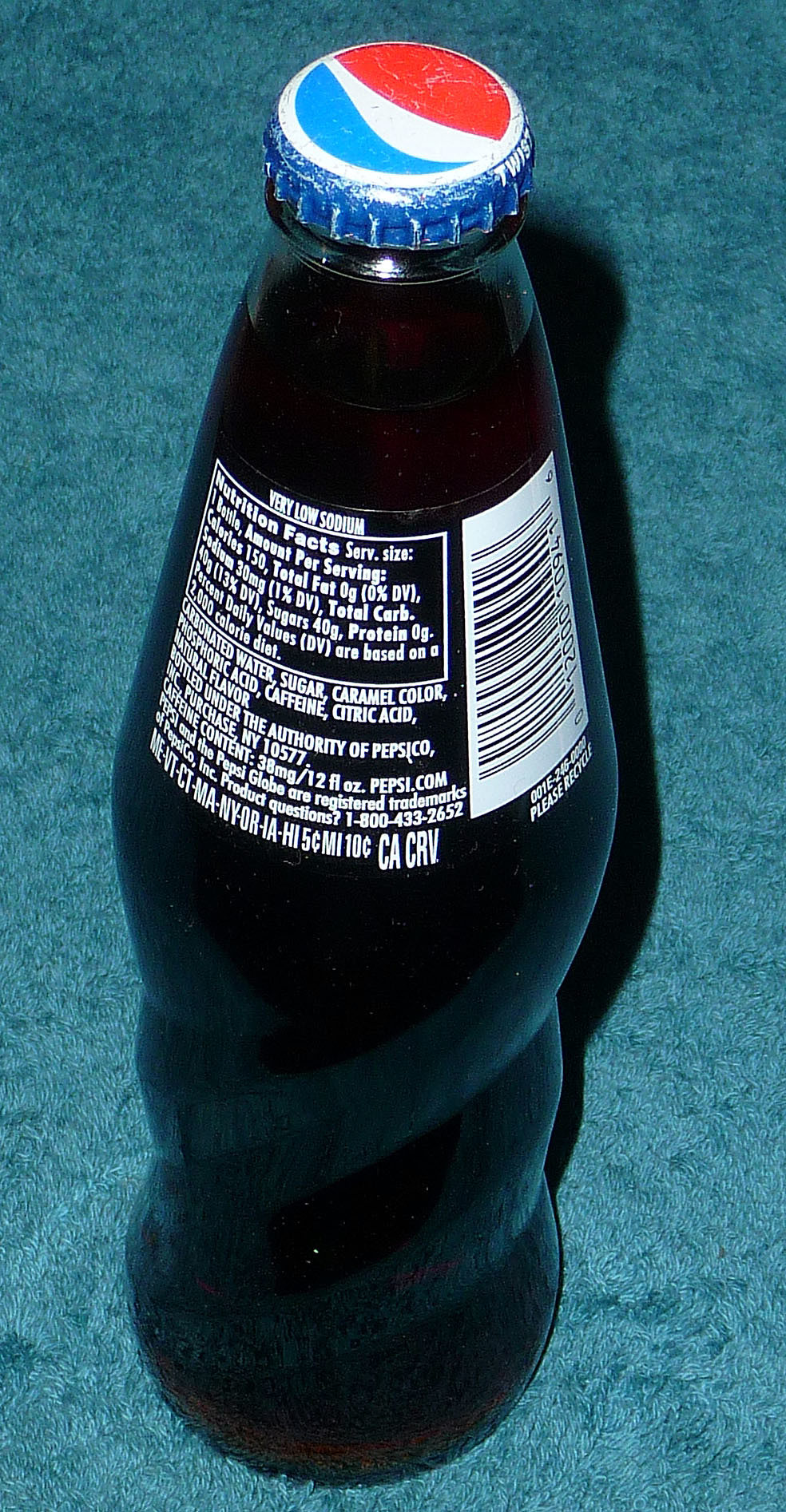Caption: 

A sealed bottle of Pepsi is prominently displayed, boasting its classic packaging. The dark-colored bottle contrasts with an eye-catching red, white, and blue cap, adorned with the iconic Pepsi logo. The label highlights "Very Low Sodium" and provides nutritional information, indicating zero grams of protein and a breakdown of ingredients including water, sugar, caramel color, caffeine, and citric acid. The product is noted to be under the authority of PepsiCo, California. The bottle rests on an aqua blue rug, creating a vibrant backdrop that emphasizes the product's distinct features. The label also includes a UPC code, though it is not clearly visible. The image captures the essence of an unopened, refreshing bottle of Pepsi, ready to quench your thirst.